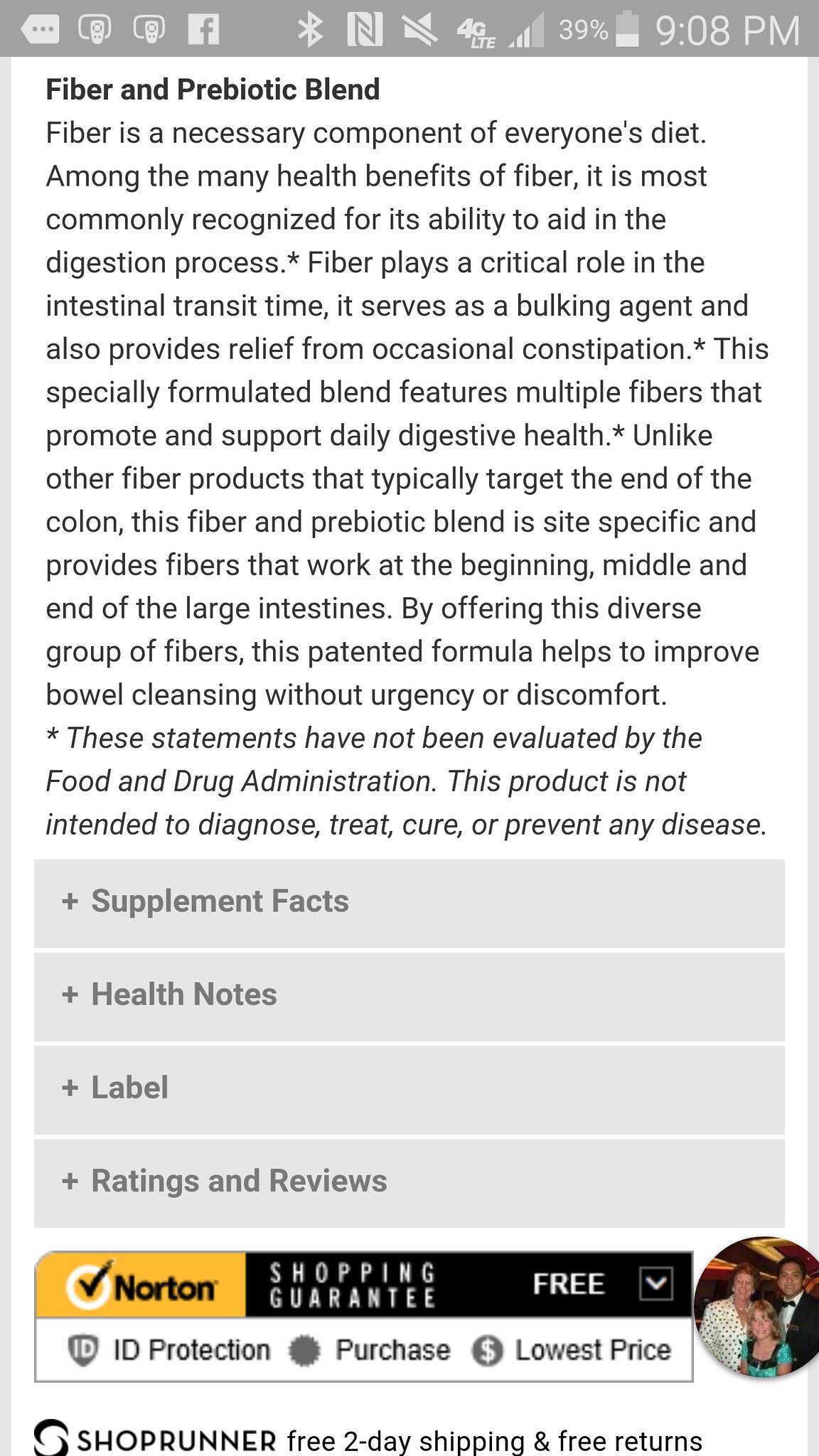The image is of a vertically oriented rectangle bordered by a light to medium gray gradient along the sides. The top section of the rectangle is framed by a thicker, slightly darker gray bar. The bottom portion lacks a distinct border, blending seamlessly into the white background of the computer screen.

In the upper gray bar, various informational icons are situated, including indicators for battery life, signal strength, time, Bluetooth connectivity, and other clickable options. The central portion of the image, set against a white background with black text, prominently features the phrase "Fiber and Prebiotic Blend." Below this headline, a brief description explains the importance of fiber in a diet.

Further down, the image contains a series of gray boxes labeled "Supplement Facts," "Health Notes," "Label," "Ratings and Review," and additional sections for detailed consumer information. Adjacent symbols include a Norton Check icon, a shopping cart, and a small circle depicting three people, potentially representing community or group benefits. The image also mentions extras like ShopRunner, which offers free two-day shipping along with free returns, enhancing the shopping experience.